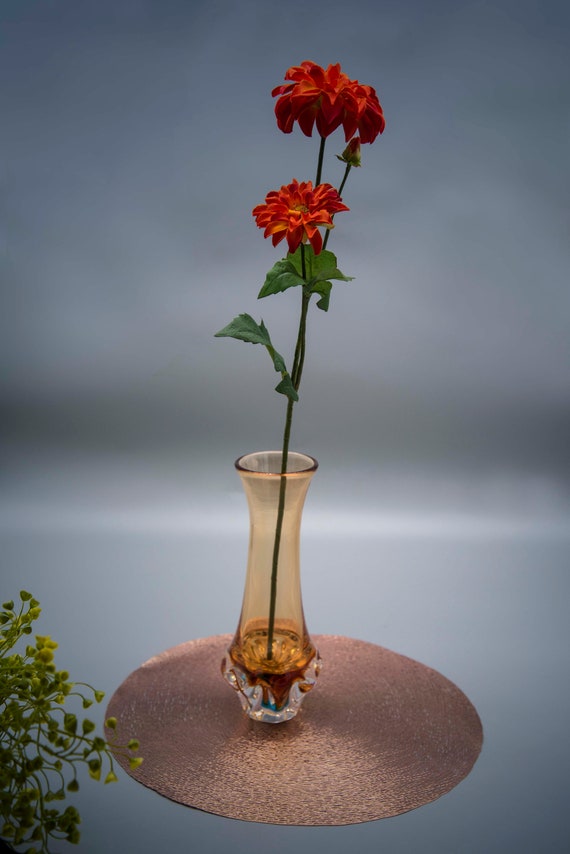Centered in this image is a small, slender vase filled with vibrant red flowers. The blossoms feature bright yellow centers, creating a striking contrast against their red petals. Emerging from the stems are lush green leaves that add a dynamic touch to the arrangement. The transparent vase, modest in size, contains a small amount of water, suggesting the flowers are freshly picked. Positioned beneath the vase is a circular mat with a shiny light purple hue, adding a subtle touch of elegance to the display. In the bottom left corner, the tops of a green plant are visible, characterized by tiny, delicate leaves that almost appear artificial. The background features a gradient of light blue to light gray tones, with an indistinct, darker object that blends into the blurry backdrop, creating a sense of depth and mystery.